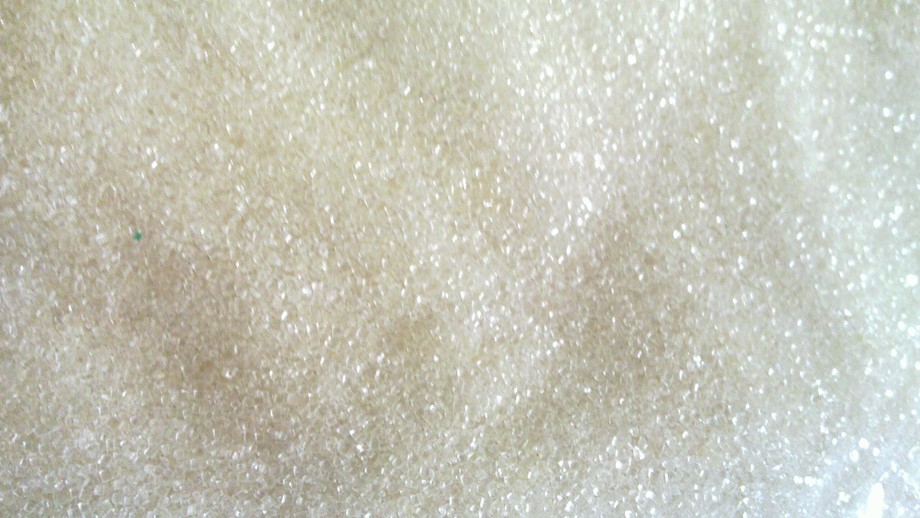The image features an uneven pile of white crystal pieces, interspersed with occasional beige and a tiny green dot near the middle left part. The crystals exhibit a granular texture and a reflective surface, especially evident towards the right side of the image. The left side predominantly shows a mix of beige and white crystals, transitioning to a shinier, more luminous appearance as you move towards the right. This illumination, likely coming from a light source located to the right or bottom right, makes the crystals appear to glimmer and shimmer, highlighting the intricate details of the finely textured material. The fabric-like quality of the pile suggests a delicate and granular makeup, with some sections appearing darker, possibly due to folds or shadows cast by the light source.